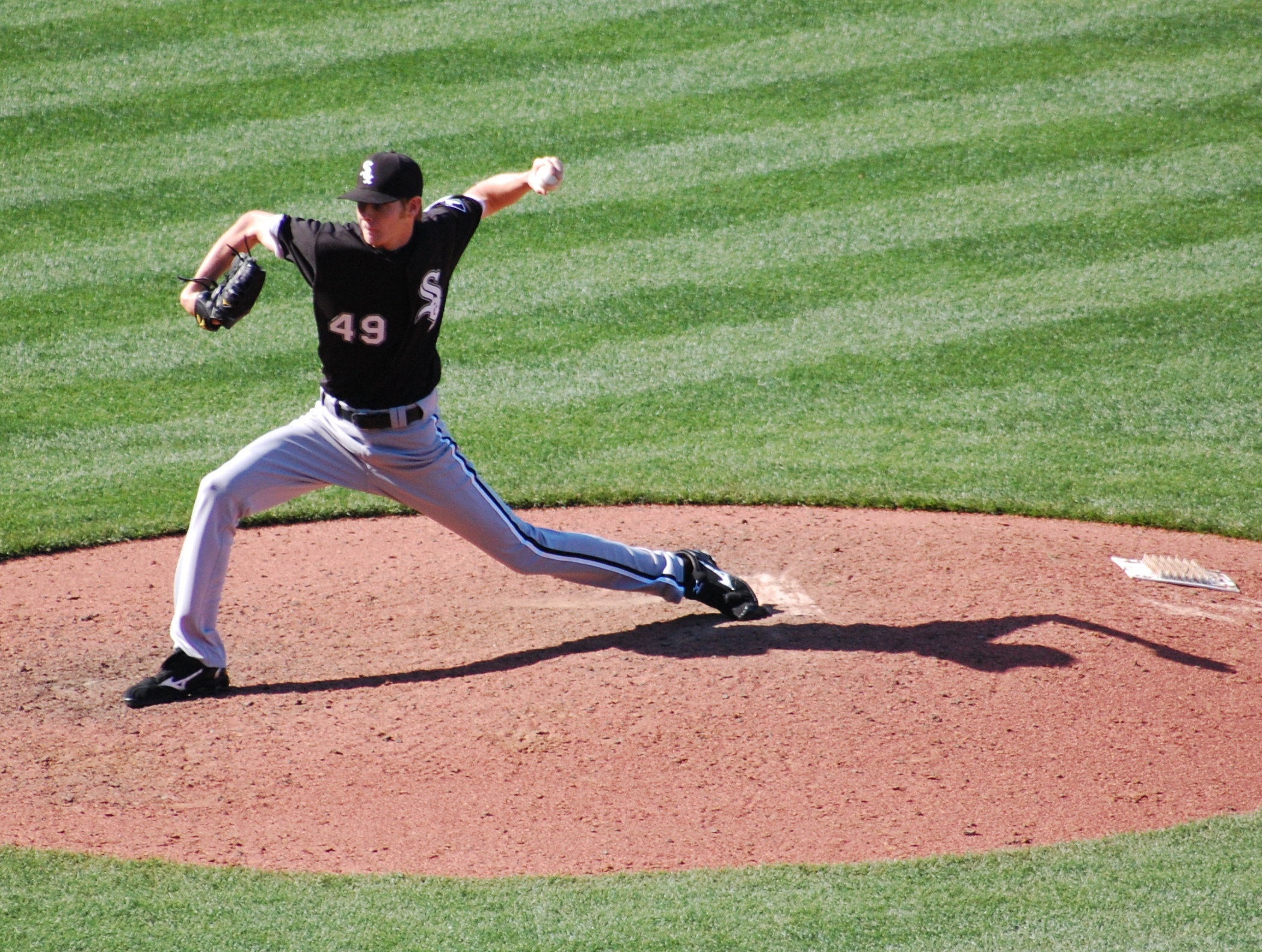In this photograph, you see a Chicago White Sox pitcher in mid-throw, captured during a game. The player, wearing jersey number 49, is clad in a black short-sleeve uniform top with white lettering and the team's "Sox" logo embroidered on both the jersey and the black cap. His pants are light gray with black and white stripes running down the sides, secured by a black belt. He is also wearing black and white cleats. The player's left arm is stretched back, holding the ball, while his right hand, fitted with a black glove, is positioned forward. His stance reflects the intensity of his pitching motion, with his left leg extended far behind and his right leg bent and positioned closer to the grass, while he stands on a mound of circular brown dirt. The sunlight glistens off his back, indicating it is a bright, sunny day.